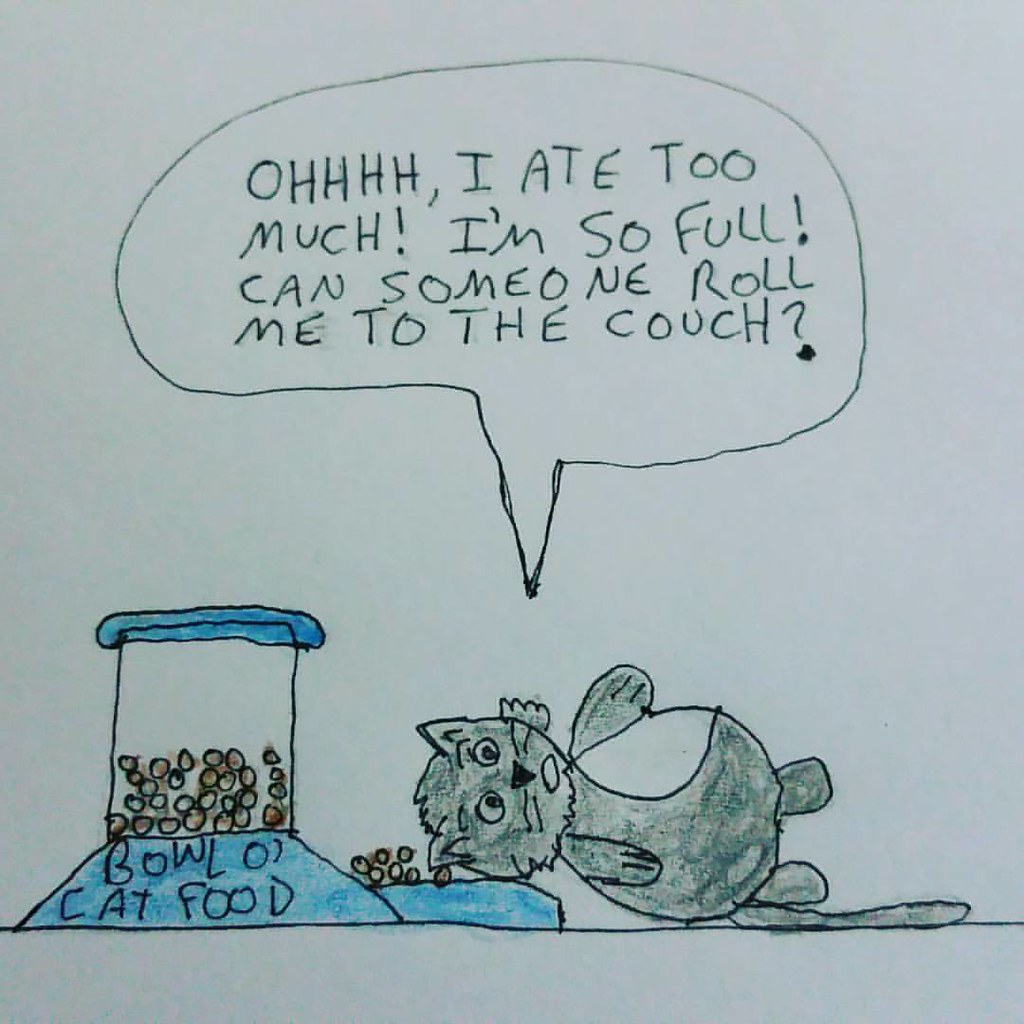A child's crayon drawing is presented on a standard white printer paper. The central focus is a blue cat feeder filled with brown cat food, clearly labeled "bowl of cat food." Next to the feeder is a plump, gray cat, depicted as lying down with its head resting on the feeder. Above the cat, a black text bubble contains a humorous message that reads, "Ow, oh, oh, h, h, h, I ate too much, I'm so full, can someone roll me to the couch?" The entire image, including the feeder, the cat food, and the text, is created using vibrant crayon colors.